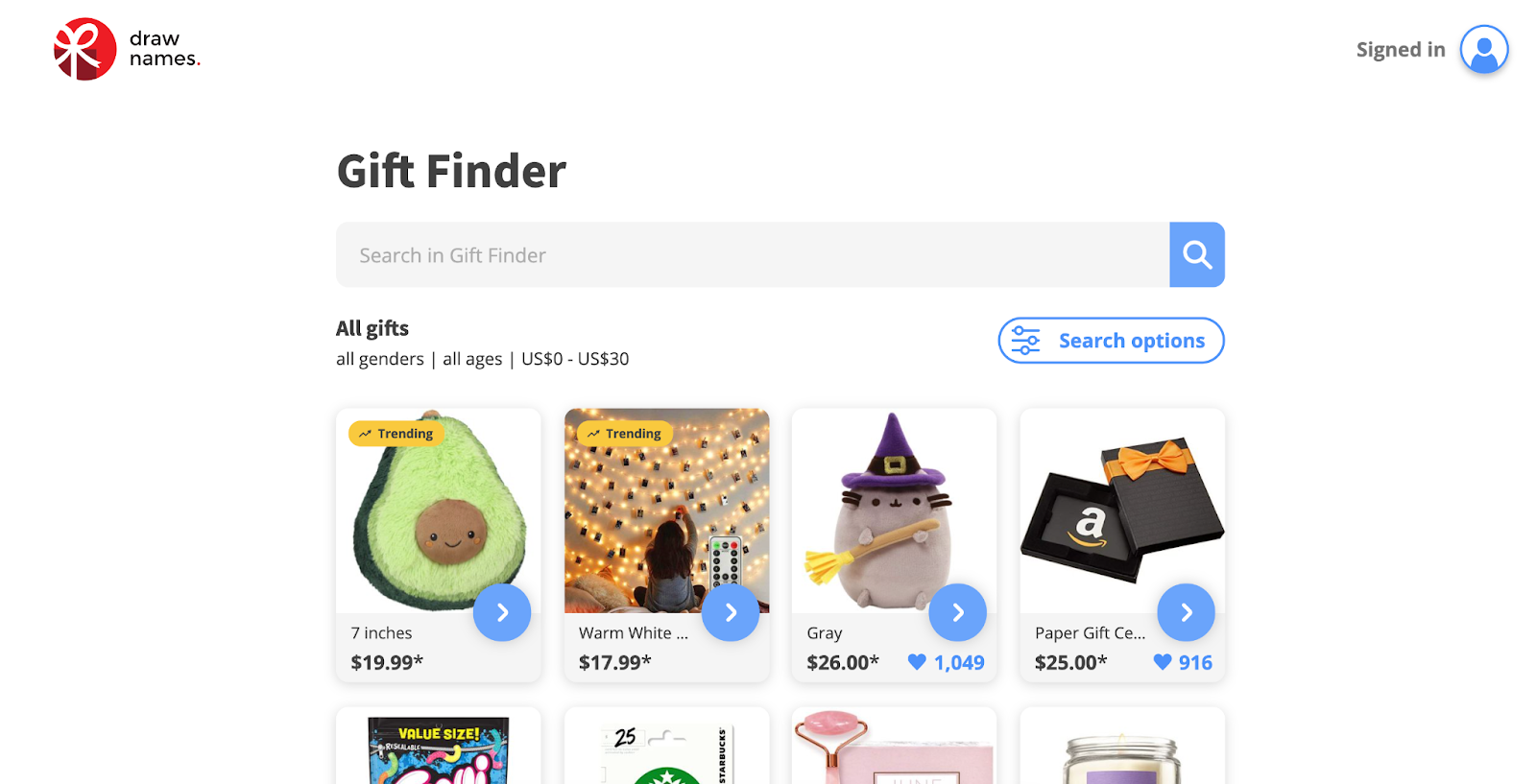In the photographed webpage, a visually engaging layout greets us. On the left-hand side, a prominent circular button stands out, adorned in shades of red, maroon, and white. This button features a graphic depicting a gift box. Adjacent to this, the phrase "draw names" is written in all lowercase using small black font. Switching our focus to the right-hand side, a "signed in" indicator is accompanied by a white circle containing a simple blue head-and-shoulders icon. 

Toward the upper section of the page, the bold text "Gift Finder" is prominently displayed. Below it, a search bar stretches across, with a blue magnifying glass icon to its right, and an input field that reads, "all gifts, all genders, all ages, US $0 to US $30".

The search options are neatly organized within an oval-shaped filter bar. Featured gifts include a $19.99 plush item: a 7-inch green avocado with a brown smiley face. Additional items include warm white string lights priced at $17.99, a whimsical gray witch cat figurine for $26, and a versatile Amazon gift card valued at $25.